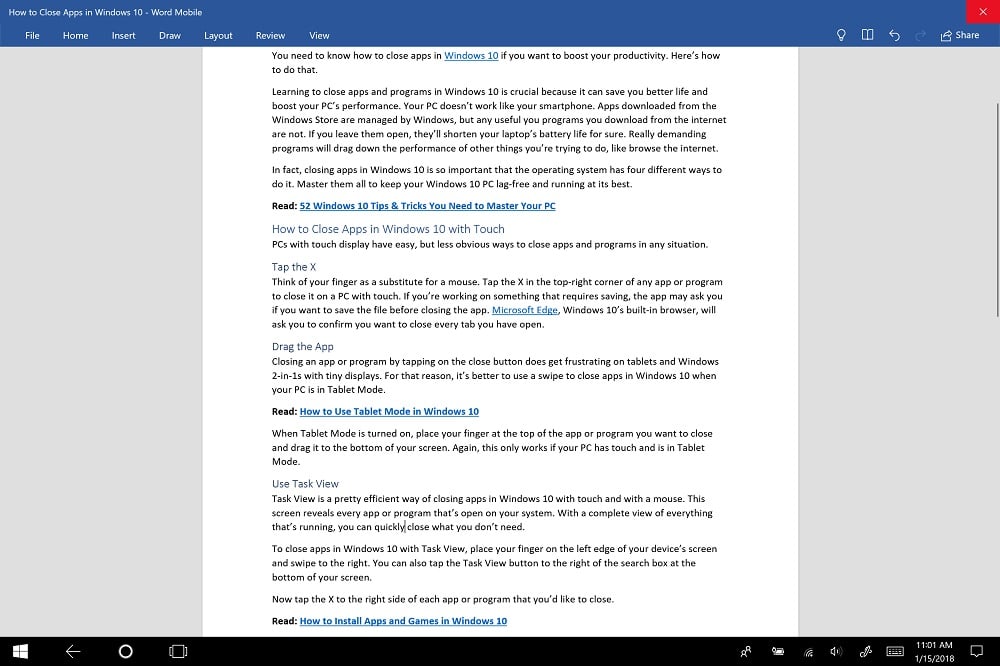At the top of the image, a dark blue banner with white text reads "How to Close Apps in Windows 10 Word Mobile." Just beneath the banner are options listed as "File," "Home," "Insert," "Draw," "Layout," "Review," and "View," accompanied by a white light bulb icon and a red square with a white X in it.

The main section of the image features a white background with black text stating, "You need to know how to close apps in Windows 10 if you want to boost your productivity. Here's how to do that." Below this, there is blue, underlined text that reads, "52 Windows 10 Tips and Tricks You Need to Master Your PC."

Further down, blue text indicates, "How to Close Apps in Windows 10 with Touch." Following this, additional black text explains, "PCs with touch display have easy but less obvious ways to close apps and programs in any situation."

Towards the bottom, blue, underlined text says, "How to Use Tablet Mode in Windows 10." Directly underneath, black text reads, "When Tablet Mode is turned on."